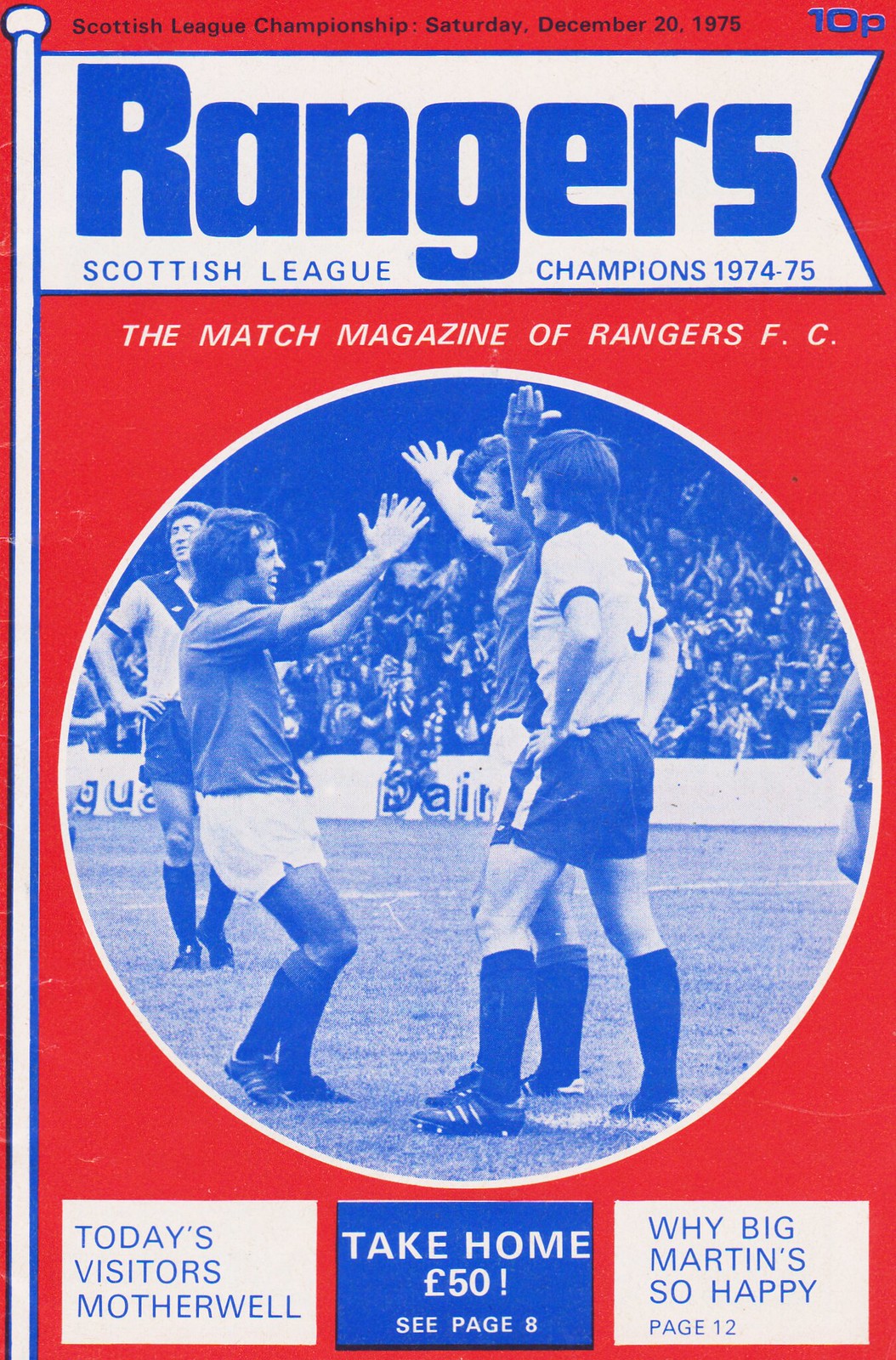The cover of this vintage sports magazine showcases a vibrant red background with a prominent circular photograph at its center, tinted in blue and white hues. The photograph captures a jubilant moment on the football field where three players are celebrating: one on the left with his arms outstretched and slightly squatting, another facing him with both hands raised in triumph, dressed in dark shirts and white shorts, and a third player with long, shaggy hair, smiling in a white shirt numbered '3' and black shorts with a white stripe. The background also reveals an enthusiastic crowd and another player.

Across the top in black text, it reads "Scottish League Championship Saturday, December 20, 1975,” with the cost “10P” printed in blue in the upper right corner. Below this in bold blue text, it states "Rangers Scottish League Champions 1974-75,” followed by "The Match Magazine of Rangers FC" in white. The left side features an illustration of a flagpole with a white banner that reads "Rangers" in bold blue letters.

Along the bottom of the cover are three distinct boxes: a white box with blue text announcing "Today's Visitors, Motherwell," a blue box with white text exclaiming "Take Home 50 Pounds! See page 8," and a white box with blue text that reads "Why Big Martin's So Happy, page 12."